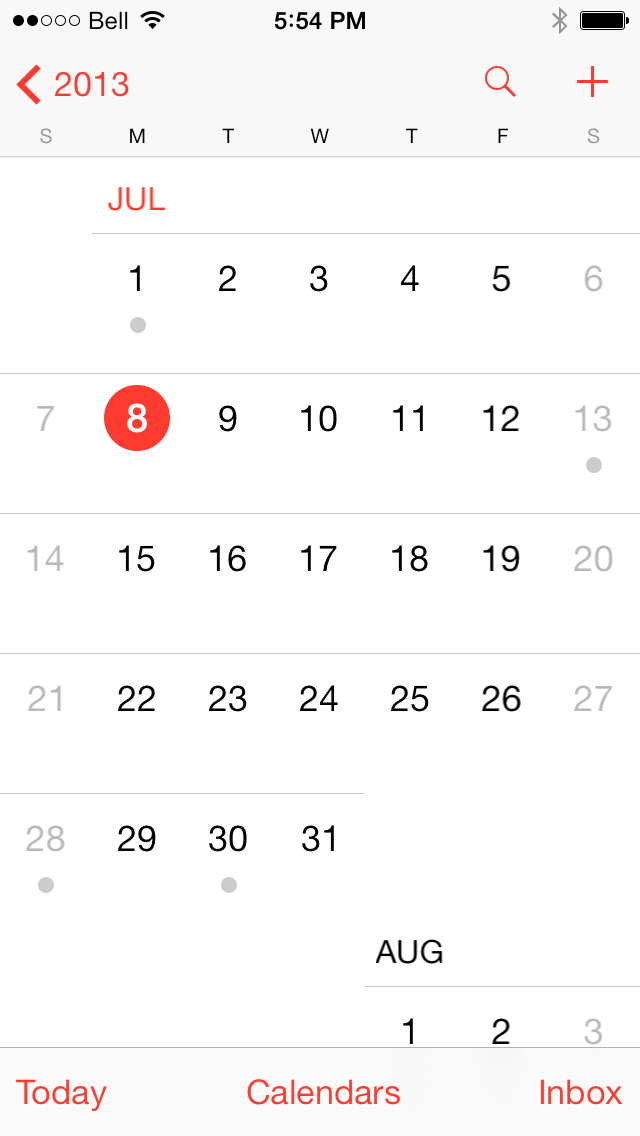A detailed screenshot of a calendar interface is displayed. At the very top of the screen, there are two out of five filled circles indicating signal strength, and a label that reads "Bell" next to the Wi-Fi symbol. The middle of the top bar shows the time as 5:54 PM. On the right side, there is a Bluetooth symbol and a fully charged battery icon.

Beneath this, there is a red left-pointing arrow on the left side, next to the year "2013." On the right side, there are icons of a magnifying glass for search and a plus symbol for adding events. The days of the week are displayed in an abbreviated format starting with Sunday (S-M-T-W-T-F-S).

Under the letter "M" for Monday, the month "JUL" is written in red, representing July. The main calendar display is for the month of July, with the current day, the 8th, highlighted. The numbers 1, 13, 28, and 30 each have gray dots below them, possibly indicating events or appointments.

Towards the bottom, the upcoming month "AUG" is displayed in black writing, with the first three days of August visible: 1, 2, and 3. At the very bottom of the screen, there are three options in red writing: "Today" on the left, "Calendars" in the middle, and "Inbox" on the right.